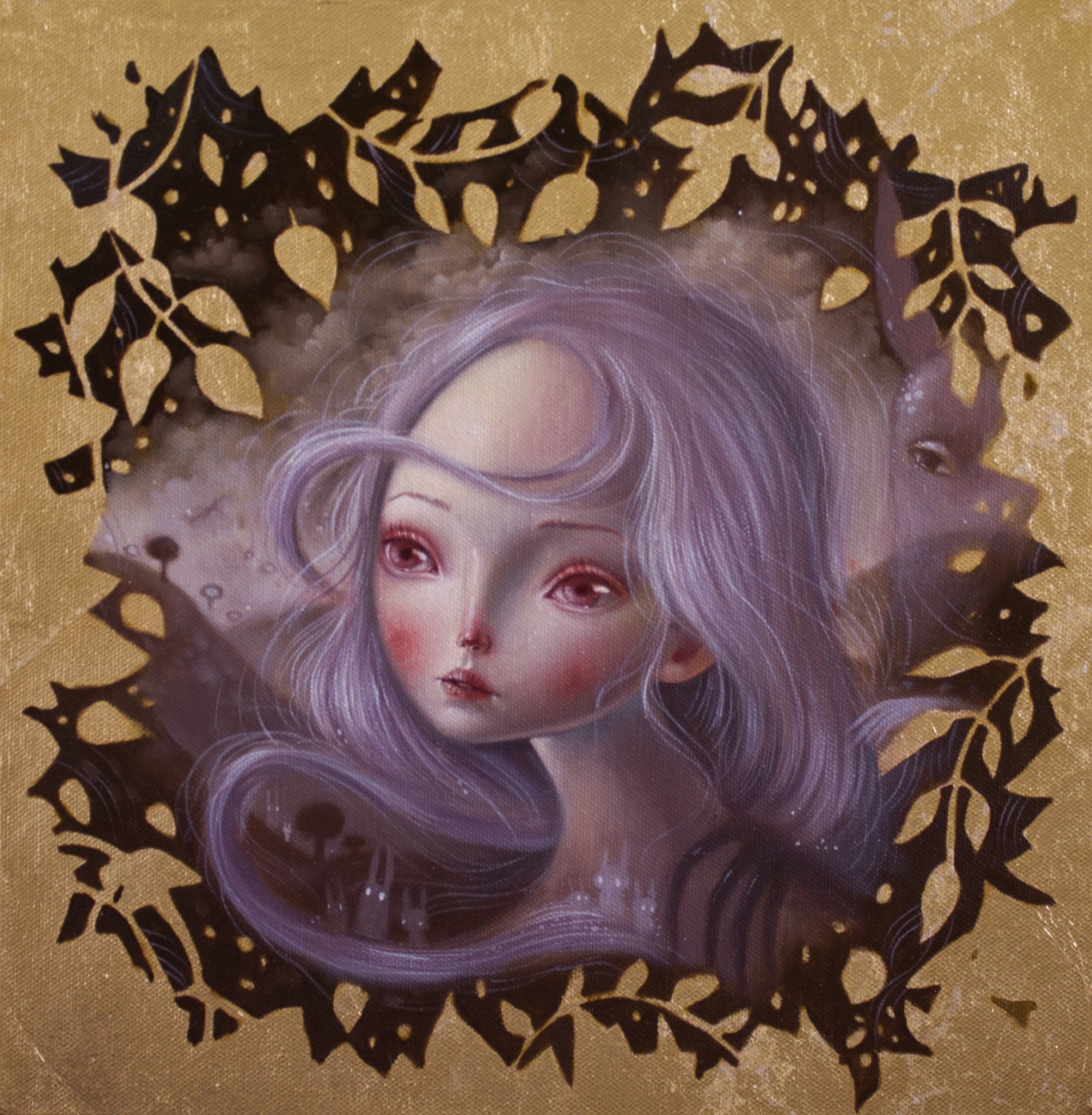This detailed painting or drawing portrays a young woman with long, shoulder-length, light violet-purple hair, with a strand elegantly crossing her forehead. She has large almond-shaped eyes, thin eyebrows, a very thin nose, thin pink lips, and blushed pink cheeks. Her expression is serious, her mouth firmly closed as she gazes slightly away to her right, adding a subtle sense of introspection. The background features a light brown backdrop adorned with intricate black decorative elements resembling emblems or squiggles. The entire image, devoid of any text, is richly colored with hues of tan, black, purple, red, and pink, and the woman is centrally positioned, making her the focal point of this seemingly hand-created or digitally crafted artwork.